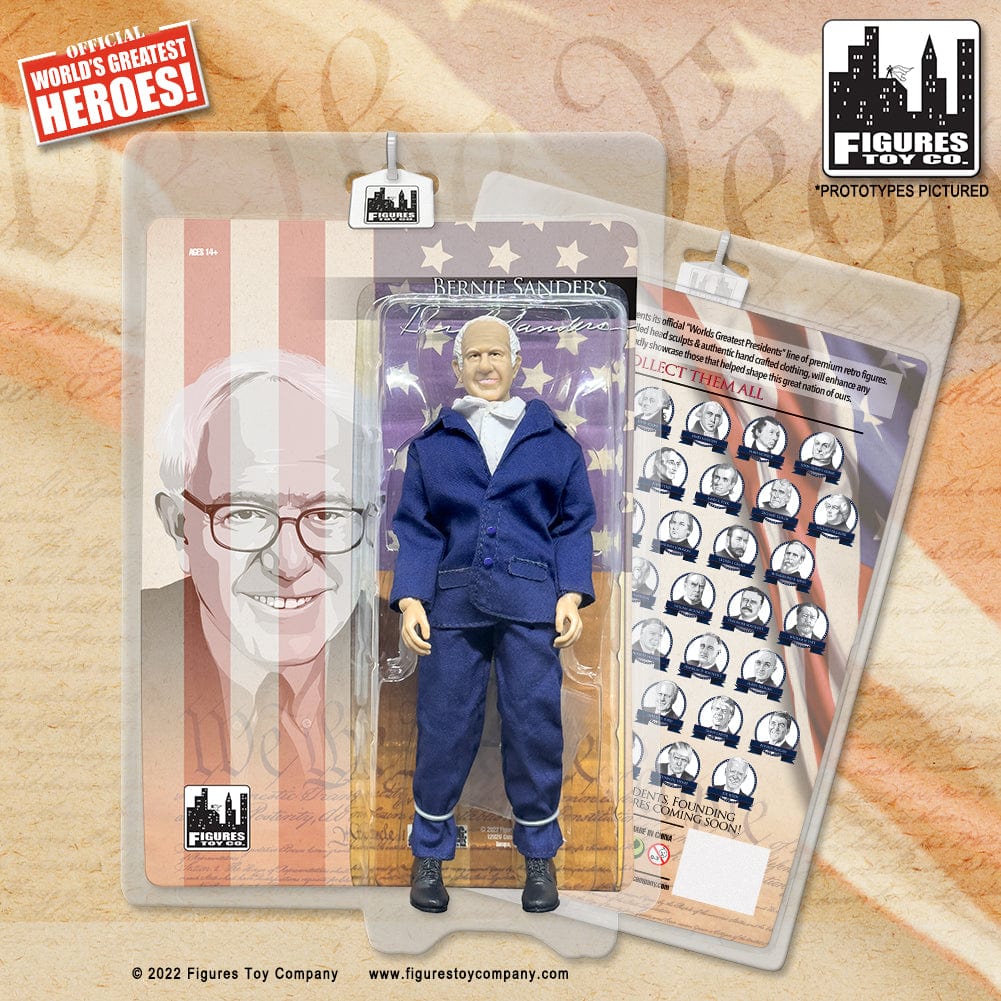The image showcases a detailed action figure prototype of Bernie Sanders, created by Figures Toy Company, which is part of their "Official World's Greatest Heroes" series. Bernie Sanders, former Democratic candidate and current Independent, is depicted in a blue suit with matching pants, a white dress shirt underneath, and black shoes. His white hair is slicked back, and he is smiling. The action figure notably does not wear glasses, unlike the side illustration on the packaging, which shows Bernie Sanders in a colorized version of his official Congress portrait. The transparent packaging features an American flag background, with a red label in the top left corner that reads "Official World's Greatest Heroes," and top right corner marking "Figures Toy Co. Prototypes Pictured." The base of the packaging indicates "2022 Figures Toy Company" along with their website, www.figurestoycompany.com. The back of the packaging includes an image that appears to be a pictured list of U.S. Presidents in black and white, set against a backdrop that might include text from the Constitution.